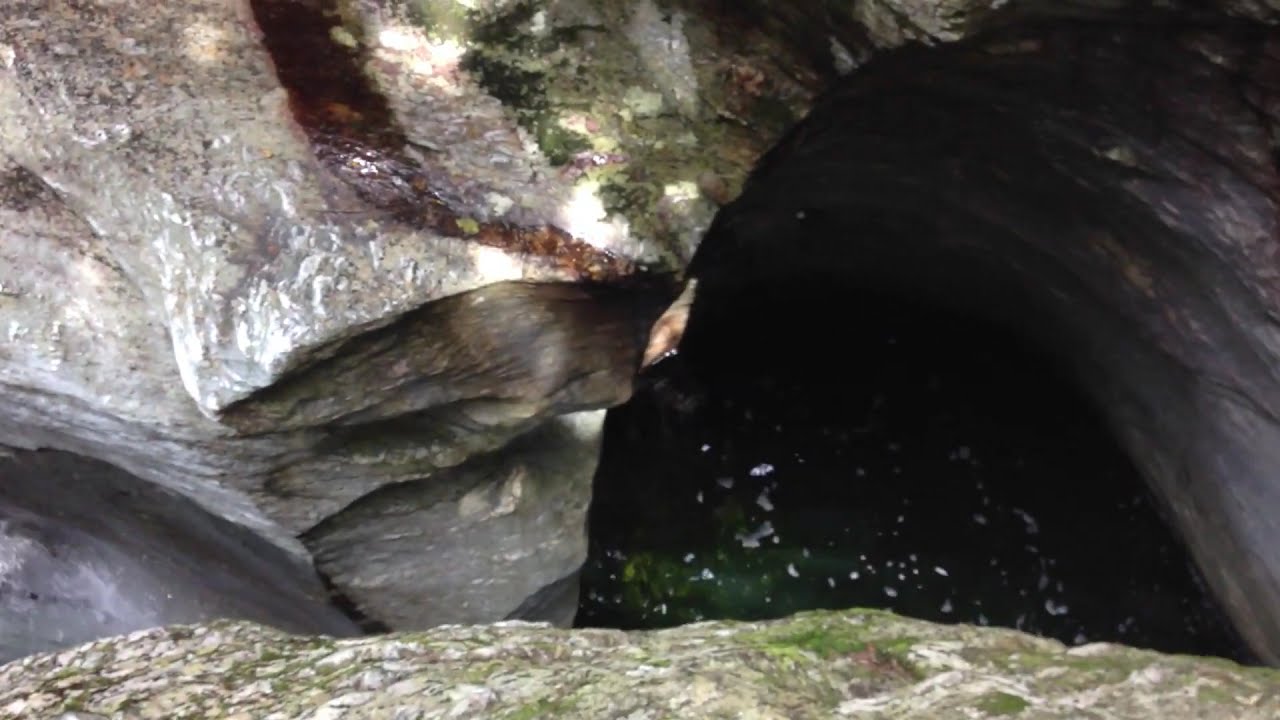The photograph captures the dramatic interior of a cave from an elevated perspective, showcasing a remarkable rock formation with an archway resembling a semicircle. This cave-like structure, adorned with a mix of grey and white hues and streaks of brown due to mineral buildup, is enhanced by the presence of moss and algae, contributing vibrant green touches to the scene. The rock surfaces, appearing wet and moist, highlight the damp environment. At the bottom of the image, a stream of greenish, murky water flows gently, displaying subtle waves and particles suspended within it. Bright green moss prominently covers a slab of rock in the foreground, suggesting the high moisture content in the area. Sunlight filters through the cave opening, illuminating parts of the cave and accentuating the textural details of the rocky walls and the stream below.